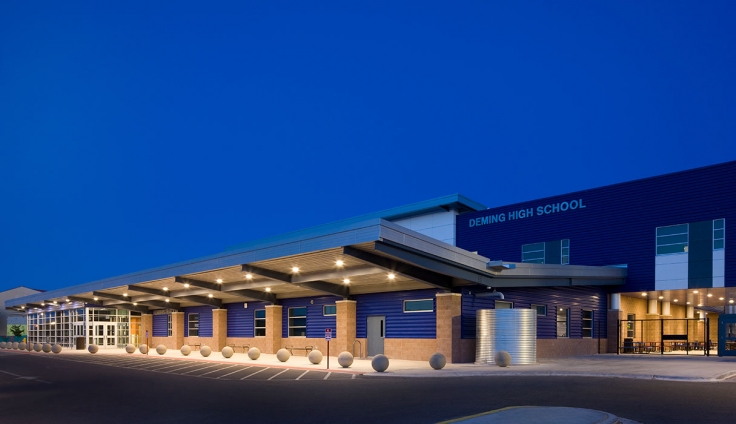This photograph captures the front view of Deming High School during the early evening or nighttime, under a dark blue sky suggesting the recent descent of the sun. The architecture features a modern design with a roof extending over the sidewalk, forming an awning that stretches from the middle to the left side of the building. Illuminated by bright LED lights, the entrance and walkway are distinctly visible. Along the ground in front of the school, there are large, spherical concrete barriers. At the top of the building, bright text reads "Deming High School," which is set against predominantly brick walls. On the bottom right side, there are glass doors and windows revealing the lit hallway inside, adding a welcoming glow to the scene. The school also includes a driveway and parking area near the entrance, facilitating loading and unloading.